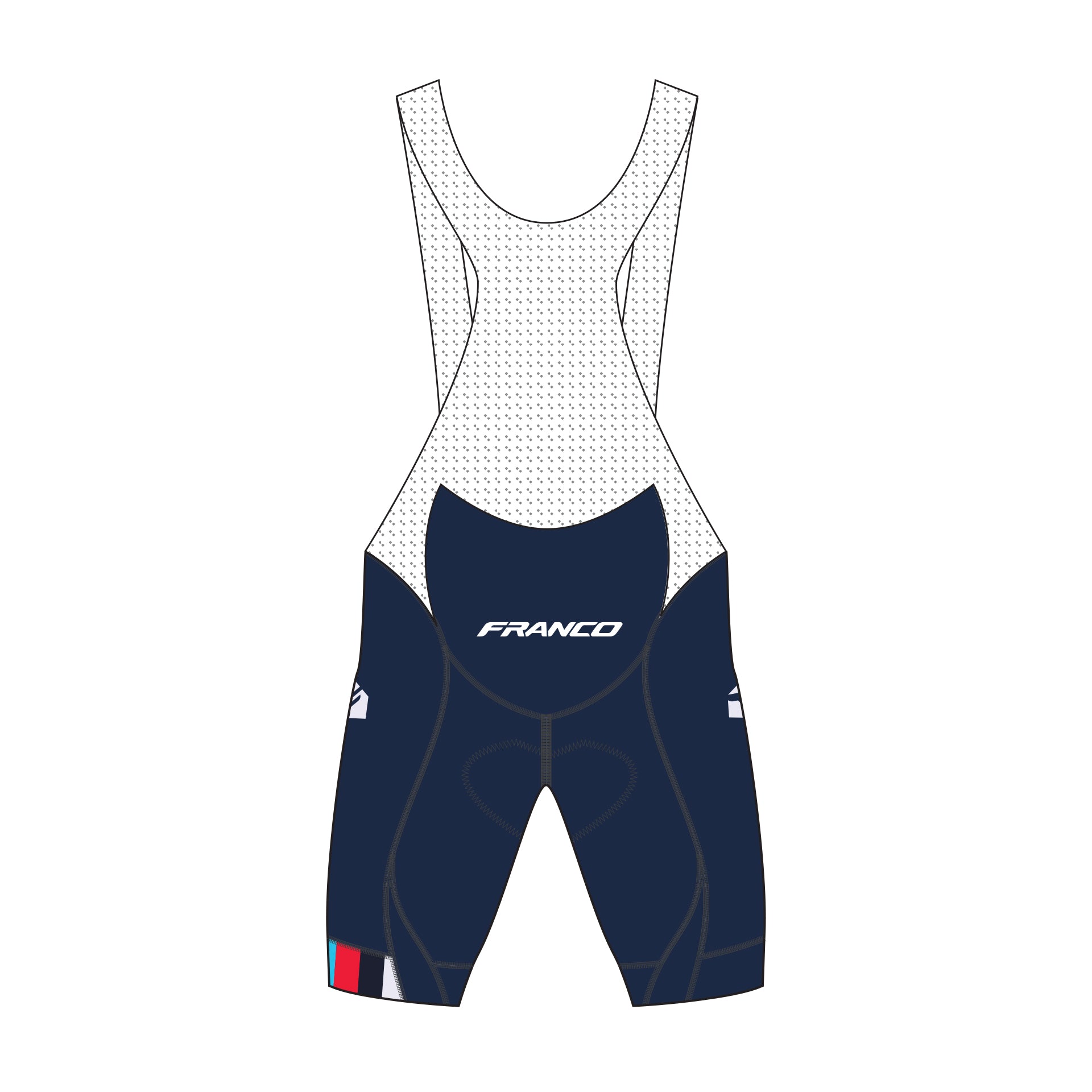The image is a detailed, drawn depiction of a cycling bib short, viewed from the rear. The upper part of the garment features white suspenders with a black check pattern, and the bib design extends over the shoulders. The primary body of the bib shorts is black Lycra, adorned with seam lines that curve along the thighs, enhancing the fit. At the waistline, the word "Franco" is prominently written in white on the butt pad. The lower-left leg sports a distinct band featuring the colors white, red, and green, potentially indicating a brand or team affiliation. Additionally, there are white flashes around the hip area.